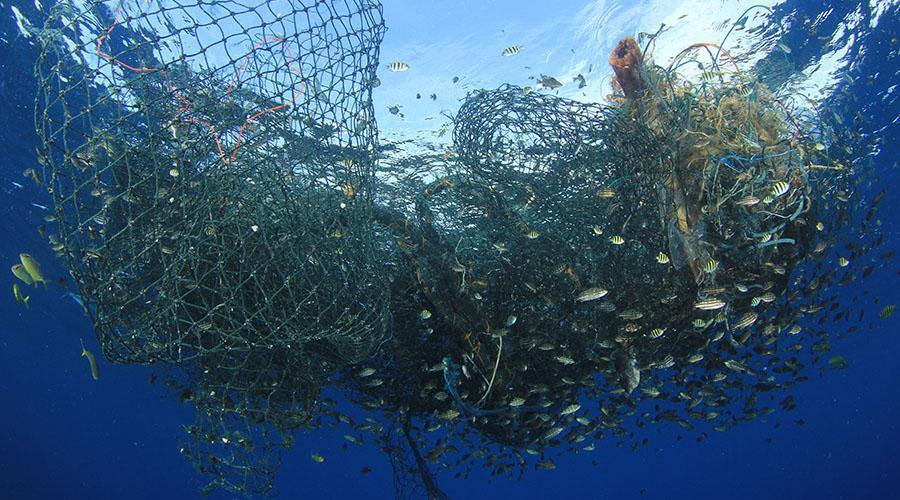The photograph captures a tangled green nylon fishing net cast off into the ocean, ensnaring various driftwood resembling brown branches, as well as an assortment of green sea life. Swimming around this entangled mass are small, disc-shaped fish in hues of green and white, as well as a school of yellow fish hovering on the left side, all amidst a dark blue, murky water. The net, taking up about two-thirds of the image, appears severely tangled and cluttered with random debris including ropes, additional plastic pieces, and strings in red, blue, and tan colors. There is something red protruding from the upper right portion of the net. The photograph is taken slightly below the surface, revealing a light blue sky adorned with white clouds. Although not all fish are caught in the net, many are distressingly entangled, likely leading to their eventual suffocation or injury.